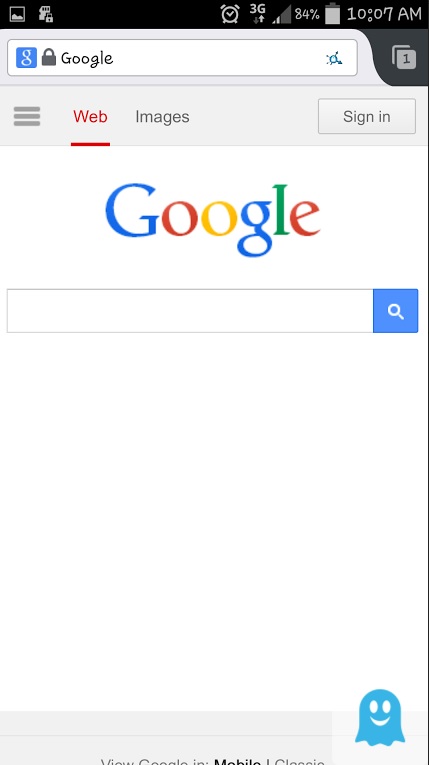This image is a screenshot taken from a cell phone.  At the top, a small black rectangle is visible, indicative of the phone's status bar. Next to it is a square icon featuring a mountain symbol, resembling a robot face. The status bar also displays '4' with a padlock symbol, hinting at a lock screen. The alarm clock icon is active, and the signal strength shows '3G' with an upward arrow, suggesting weak Wi-Fi service. The battery icon indicates 84% charge, and the time reads 10:07 a.m., all in white font.

Directly below, there's a green or blue rectangle with a white 'G' inside a padlock, followed by the word 'Google' in a white search bar. One tab is open, recognizable by three horizontal parallel lines. 'Web' is underlined in red, and adjacent to it is the word 'Images'. A sign-in rectangle features the Google logo and a blank space for entering a search query. To the right is a blue rectangle containing a white magnifying glass icon.

At the bottom of the screen, a small blue ghost icon with two eyes and a smiling face adds a charming touch.